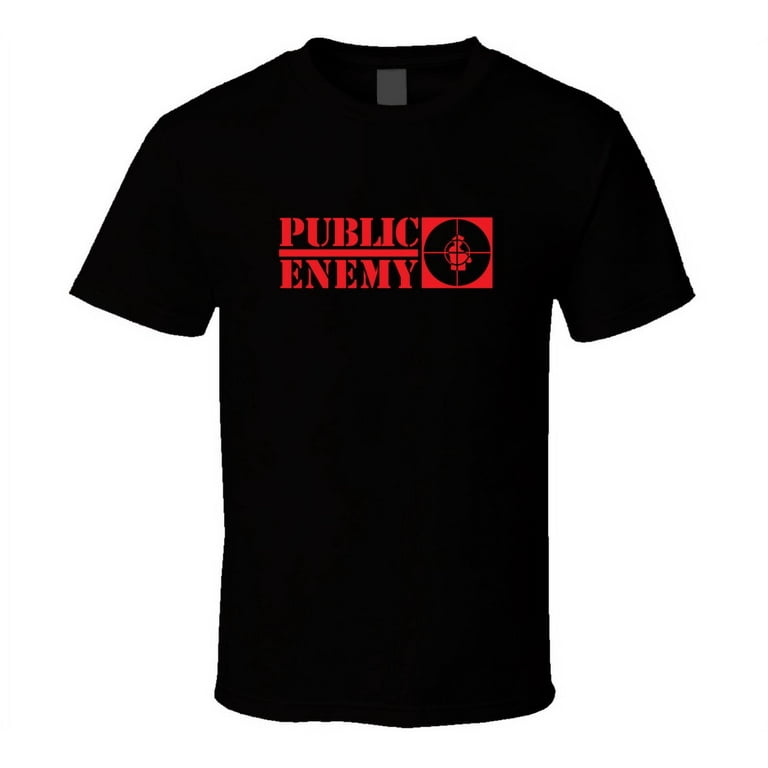This image features a black t-shirt prominently centered against a completely white background, highlighting its details. In the middle of the shirt, specifically on the chest area, there's a rectangular red logo with the bold, all-caps text "Public Enemy." Adjacent to the text, on the right side of the rectangle, is a white bullseye with a figure centered in the crosshairs, resembling a sniper scope. At the top back portion, a gray tag is visible, sewn into the collar. The shirt has a standard collar and short sleeves. Overall, the stark contrast between the black shirt and the white background emphasizes the design, making it the focal point of this potential product image.